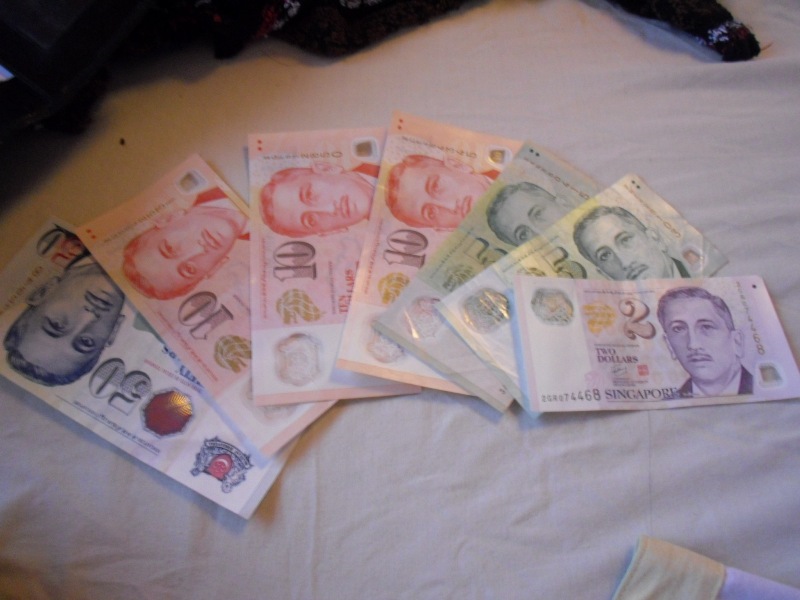In a dimly lit image, various Singaporean currency bills are displayed on a smooth, white sheet. The bills are arranged in a fan-like, semicircular pattern, extending from the bottom left corner to the bottom right corner. The bills include a $2 bill in light purple with a small moustached gentleman's portrait and "Singapore" written at the bottom, five $5 bills in a light green hue, three $10 bills featuring a pink design with hints of gold and white on one half, and a prominent $50 bill with a silvery grey and red accents. The bills collectively show the detailed engravings and colors representing Singaporean currency, set neatly against the simple white backdrop, with a section of black and light whitish visible at the top right corner of the frame.